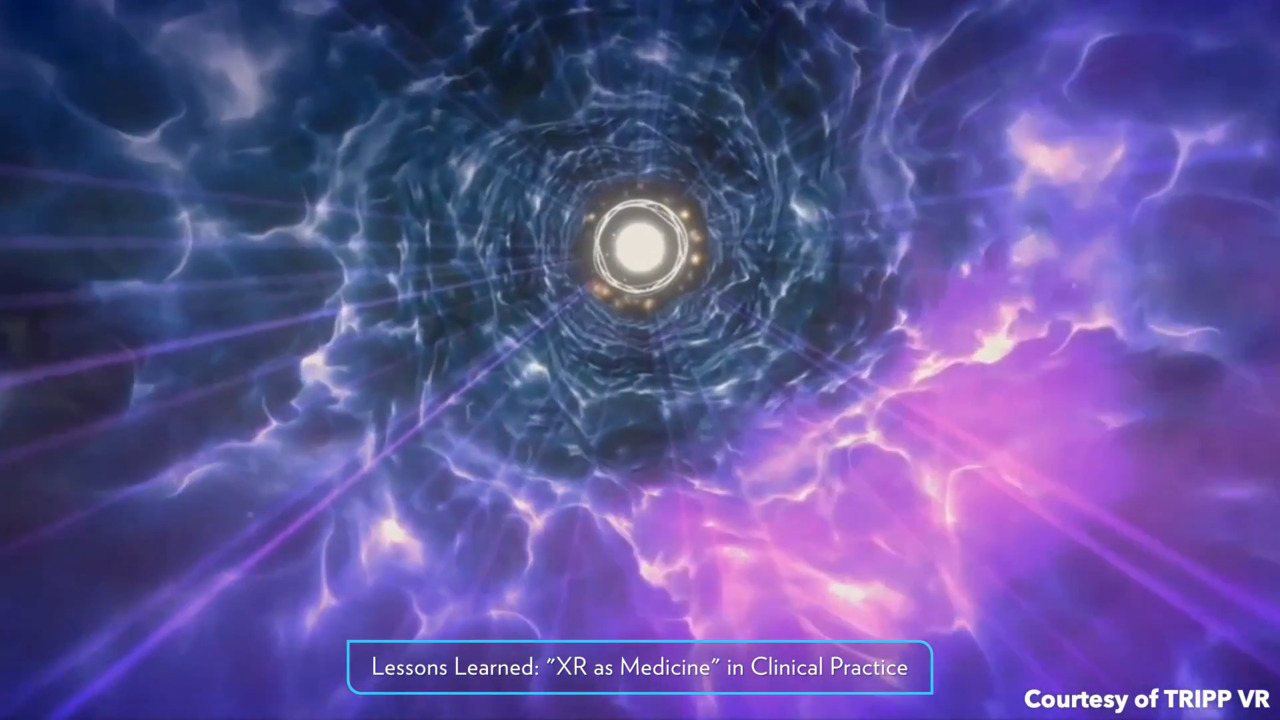This intricate image captures a mystical, tunnel-like scene with a bright, radiant light at the center, giving the impression of an exit in the far distance. The central bright light is surrounded by concentric layers: initially, a black outline, followed by four strands of yellow light, another black boundary, and then an outer ring of dark blue transitioning to purple as it extends outward. Enclosing this vivid core is a tube-like structure composed of smoky, cloud-like formations filled with dark blues and purples. These clouds, especially towards the bottom, are illuminated with pinks and purples, reminiscent of storm clouds with streaks of lightning forming a U-shape across the bottom section of the image. Rays of purple light beam outward through the scene, further enhancing the mystical feel. At the very bottom, prominently displayed in a blue rectangular box with rounded edges, is the white text that reads, “Lessons Learned: XR as Medicine and Clinical Practice.” In the bottom right corner, additional white text credits the image to "Courtesy of Trip VR."